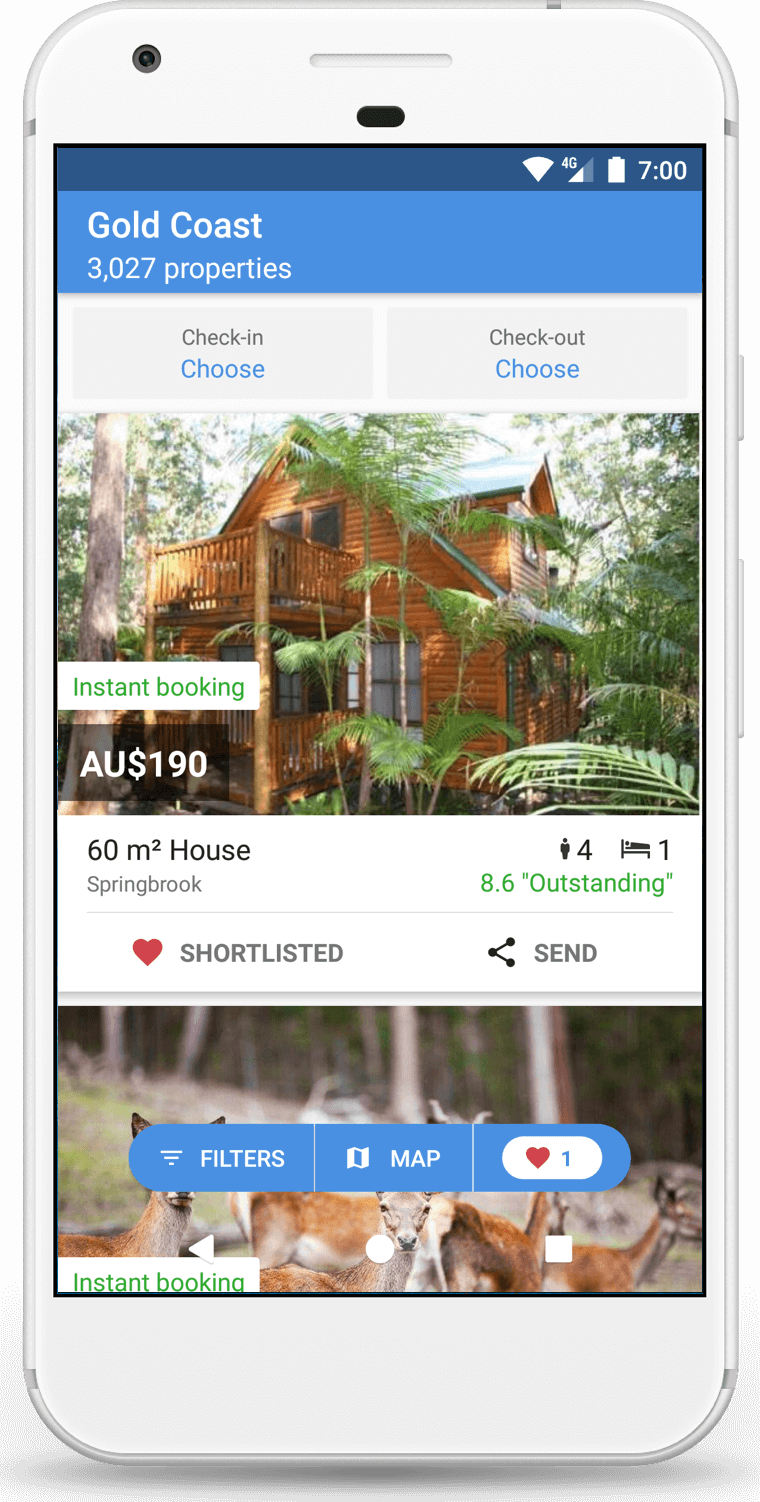The screenshot displays a smartphone with a clear white border around it, showing the current time as 7 o'clock. The phone has about 2 out of 4 bars of signal strength. 

At the top of the screen, there's a dark blue banner displaying various icons. Below this banner, a larger light blue section, approximately three times its size, contains white text that reads "Gold Coast, 3027 properties." 

Beneath the blue section are two buttons: "Check in" on the left and "Check out" on the right, both accompanied by blue hyperlinks labeled "choose." 

Following this, an image of a rustic, medium-sized wooden house is shown. The house features a charming balcony both at the top and the bottom levels, with the lower level having a deck constructed from large lumber pieces resembling tree trunks. 

Below the image, the text describes the property as a "60 square meter house, Springbrook," followed by two buttons labeled "Shortlisted" and "SIN." Additionally, there's a ranking of "8.6, outstanding."